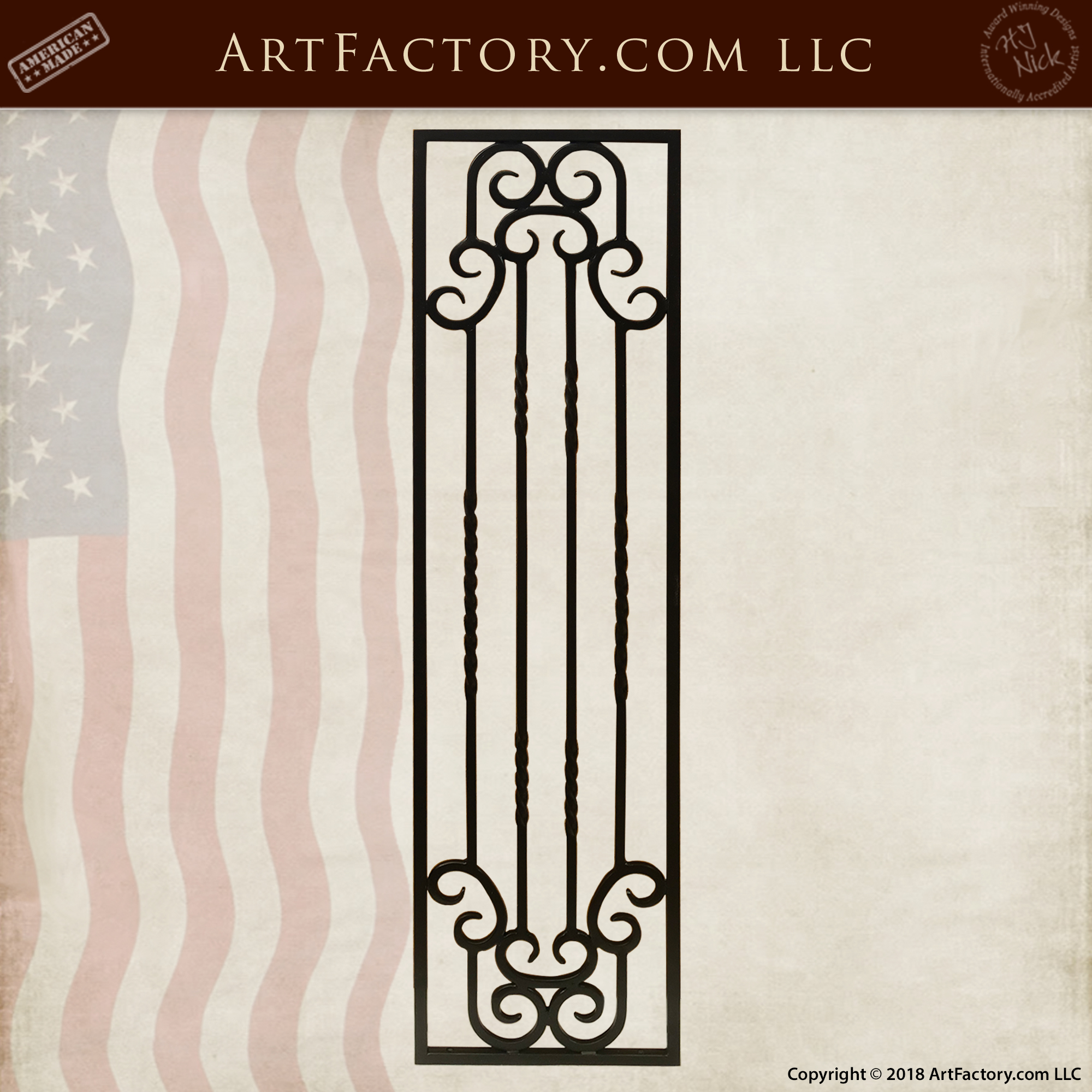The photograph showcases a tall, narrow, rectangular window grill, likely constructed from black iron. The grill features four vertical lines extending almost from the top to the bottom and includes ornate, curved decorative elements at both ends. At the top of the image, the text "artfactory.com LLC" is prominently displayed, while the upper left corner features the phrase "American Made," accompanied by a faint, background American flag. The image also notes "Copyright 2018, artfactory.com LLC" in the lower right corner. The grill, resembling an elegant outdoor gate or decorative art piece, has a formal aesthetic, set against a subtle, textured background.